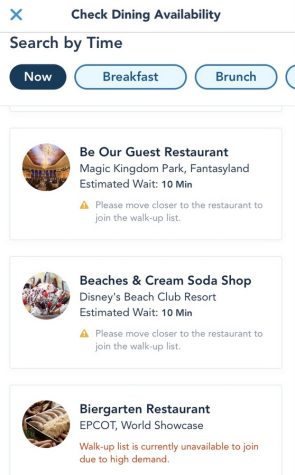This image depicts a webpage for dining reservations. The page features a clean white background. At the top left, a blue "X" icon is visible, which likely represents a close or exit button. To the right of the icon, there's the heading "Check Dining Availability" followed by a thin gray line that separates the header from the search options. Below this divider, the prompt "Search by time" is displayed.

A navigation bar allows users to filter search results. The "Now" tab is highlighted in a dark blue or black color, suggesting it is the currently selected option. To its right are two lighter blue buttons labeled "Breakfast" and "Brunch," offering additional filtering options.

Under these filters, there are three rectangular tiles outlined in light gray. Each tile provides details about different dining establishments. The first tile features "Be Our Guest Restaurant," located in Magic Kingdom Park's Fantasyland, with an estimated wait time of 10 minutes and a note that advises guests to move closer to the restaurant to join the walk-up list. The second tile highlights "Beaches and Cream Soda Shop," and the third showcases the "Biergarten Restaurant."